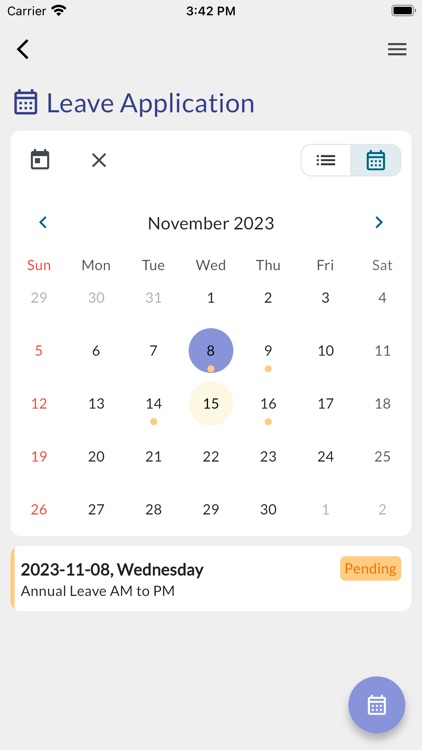The screenshot appears to be of a smartphone displaying a calendar application, taken at 3:42 PM. The top section of the screenshot features a gray background with the word "carrier" in the upper left corner, alongside three bars of decreasing length, likely indicating a Wi-Fi signal. To the right, the time "3:42 PM" is displayed prominently, accompanied by a fully charged battery icon in black.

Below this, there is a calendar interface dominated by a blue highlighting theme. The specific entry "leave application" is prominently shown in blue. The main calendar view focuses on November 23rd, with the days of the week listed at the top in a horizontal layout: Sunday (in red), Monday, Tuesday, Wednesday, Thursday, Friday, and Saturday (all in black).

Particularly notable is the date November 8th, which is highlighted in blue with a circular outline around it. Directly below, it is labeled as "2023-1108 Wednesday" and marked with the note "annual leave AM to PM pending." This indicates that the individual has scheduled an all-day pending leave on November 8th, 2023.